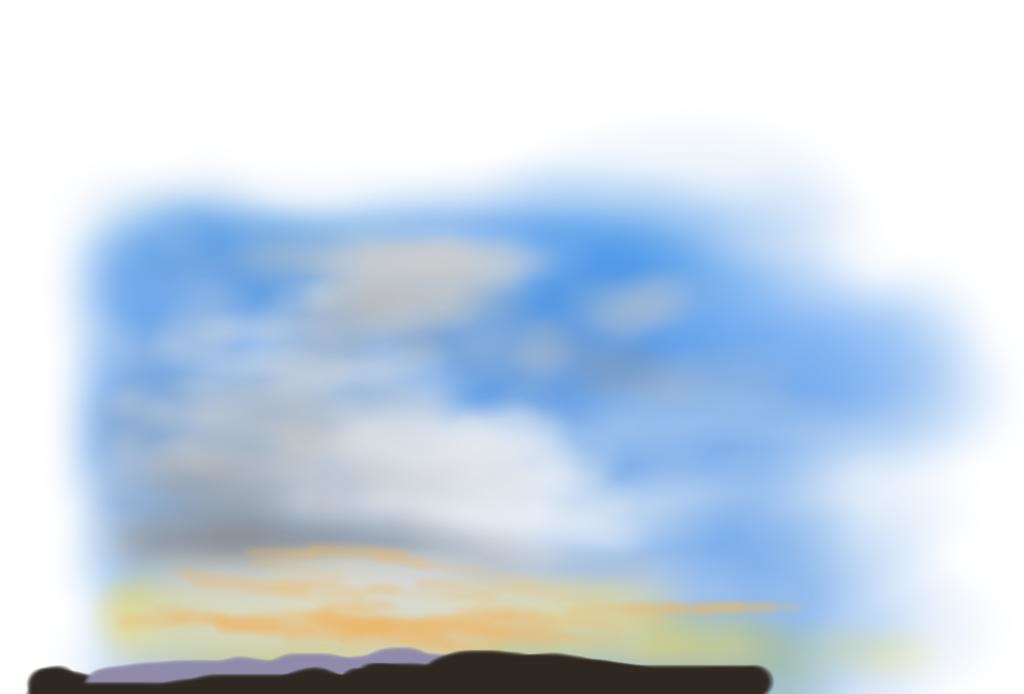The painting depicts a serene scene dominated by a vast blue sky with patches of white and gray clouds. Toward the bottom of the painting, there is a vibrant yellow sun with wavy edges, creating a harmonious blend with the sky. Hints of orange and pink are interspersed among the clouds, adding a delicate warmth to the setting. Below the sun, a subtle transition moves from faded white to light blue, indicative of the sky merging into the horizon. The bottom portion of the painting features a solid black horizontal line, suggesting the silhouette of a distant, uneven hill or rocks, with a purple shading above it. This darker area contrasts with the lighter sky above, giving the impression of a serene sunset, possibly at the beach or near a river, with a calming, ethereal quality. The entire composition is framed by a white border, enhancing the focus on the central scene.